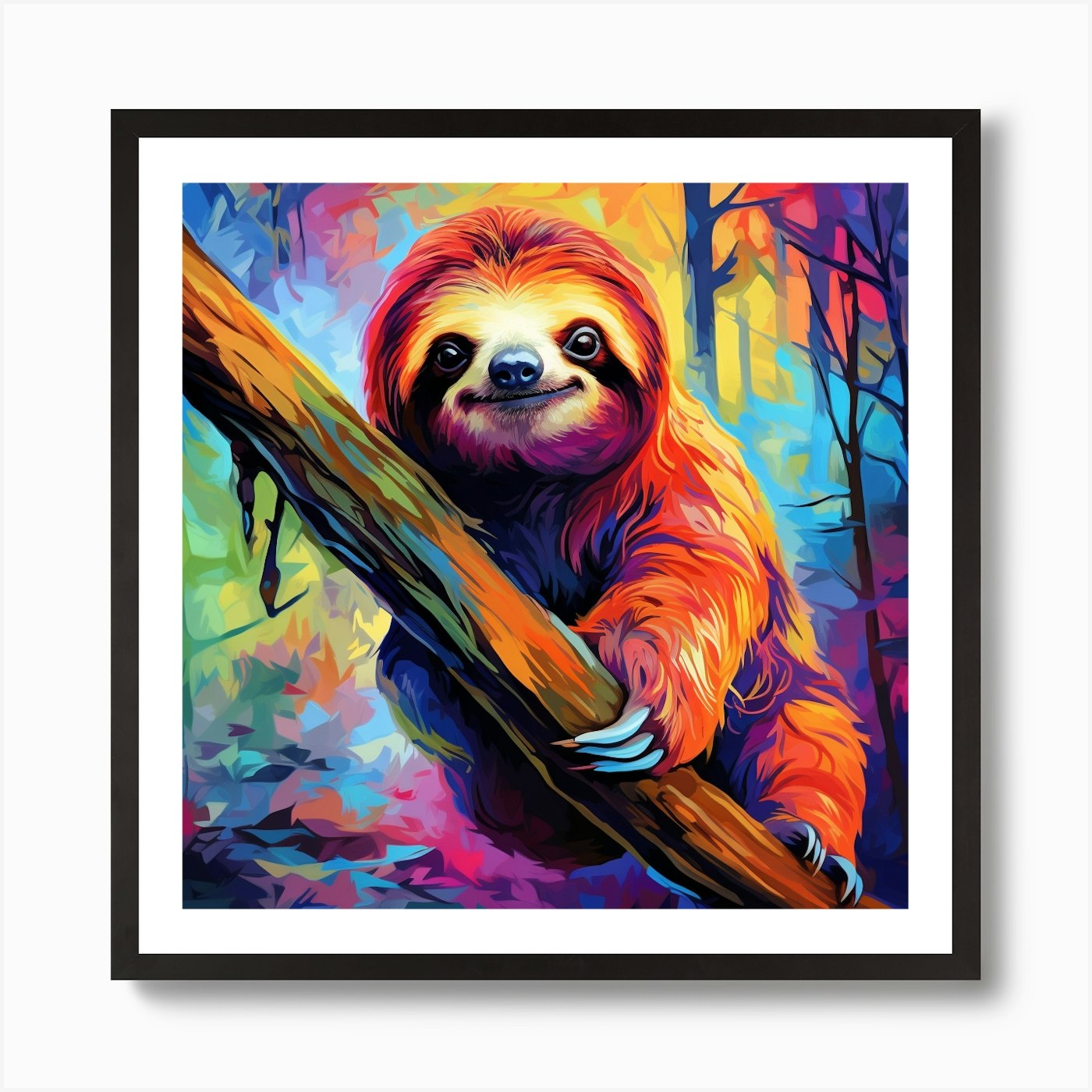The painting depicts a sloth gripping a tree branch that stretches diagonally from the lower right to the upper left corner of the canvas. This vibrant artwork, housed in a black frame with a white matting, captures the viewer's attention with its intense color palette. The sloth, adorned in an array of colors such as orange, yellow, pink, blue, and purple, is the centerpiece of the composition. Its body is long and furry, featuring expressive black eyes, a black nose, and a captivating smile. Its white claws are prominently visible, emphasizing its grip on the branch. The background is a lively mix of abstract colors, blending blues, pinks, yellows, and purple hues, interspersed with tree branches devoid of leaves. This striking and colorful scene is set against an off-white wall, enhancing the vividness of the artwork.